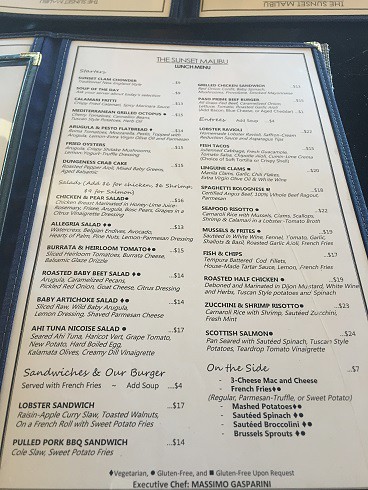This image depicts a partial view of a restaurant menu, specifically framed in a long, vertical format. The primary focus is on the lower portion of the menu, which is more in focus in the image due to the angle of the shot. The menu itself features a white main page and is encased in a blue holder, indicating the presence of additional pages. The left side of the image reveals part of the blue binder that secures the menu. The top portion of the menu displays the title "The Sunset Malibu Lunch Menu." Progressing towards the bottom of the menu, the text becomes clearer and items are more legible. At the very bottom, the menu credits "Executive Chef Massimo Gasparini," emphasizing the chef's role in curating the dishes.